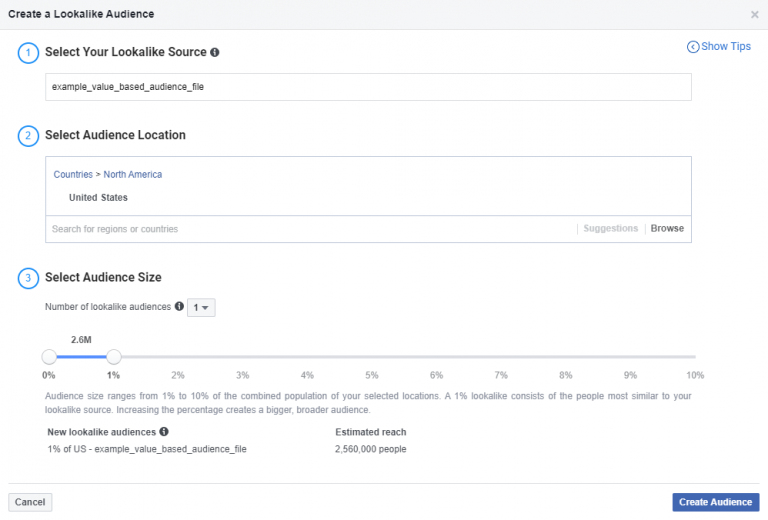**Web Page Screenshot: Creating a Lookalike Audience Detailed Breakdown**

At the top of the screenshot, there is a thin gray bar displaying the title "Create a Lookalike Audience," with an "X" button on the right side to close the window.

### Section 1: Select Your Lookalike Source
- **Indicator**: A blue circle contains the number "1".
- **Instruction**: "Select your lookalike source."
- **Icon**: An eye symbol in a black circle suggests additional information is available.
- **Tip Option**: "Show Tips" is written in blue, with a left-pointing caret indicating it's a clickable link.
- **Input Field**: The search bar contains the text "example_value_based_audience_file".

### Section 2: Select Audience Location
- **Indicator**: A blue circle contains the number "2".
- **Instruction**: "Select audience location."
- **Region Selection**: "Countries" is written in blue, and a right-pointing caret suggests expandable options.
- **Pre-selected Location**: "North America" is displayed in blue, with "United States" chosen beneath it.
- **Additional Input**: Below the selected region, there's a bar labeled "Search for regions or countries," with options "Suggestions" and "Browse" on the right.

### Section 3: Select Audience Size
- **Indicator**: A blue circle contains the number "3".
- **Instruction**: "Select audience size."
- **Number of Lookalike Audiences**: An information icon is present for further details. The drop-down menu has "1" selected.
- **Audience Size Slider**: Scale line ranges from 0% to 10%, with the range 0% to 1% highlighted.
- **Detailed Info**: Text explaining audience size:
  - "Audience size ranges from 1% to 10% of the combined population of your selected locations."
  - "A 1% lookalike consists of the people most similar to your lookalike source. Increasing the percentage creates a bigger, broader audience."
- **Specific Audience Note**: "New lookalike audiences" with an information icon. The highlighted audience is "1% of US example_value_based_audience_file, estimated to reach 2,560,000 people."

### Action Buttons
- **Bottom Left**: "Cancel" button.
- **Bottom Right**: "Create Audience" button.

This comprehensive layout guides users through the steps of creating a lookalike audience, detailing the source selection, location targeting, and audience size adjustments.